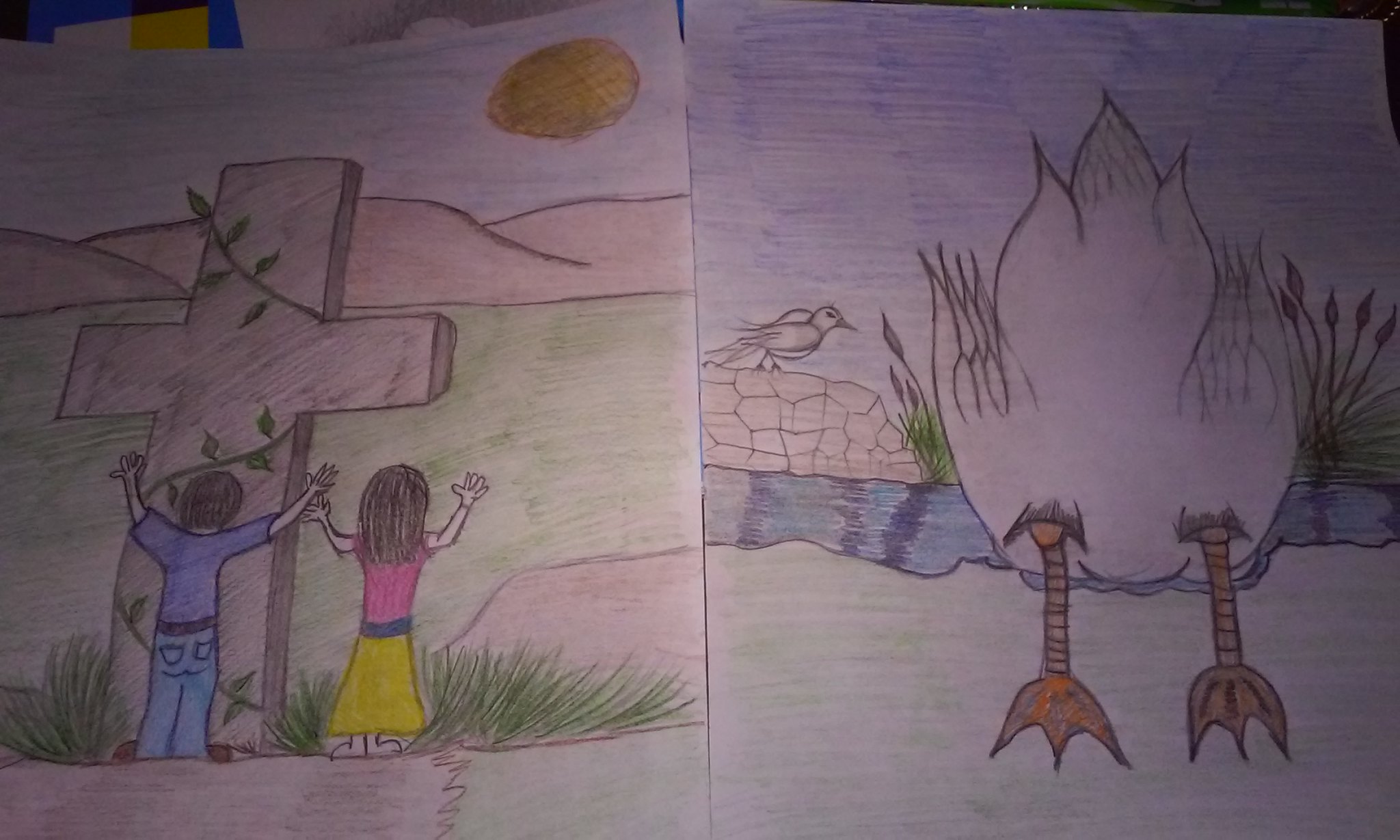The photograph captures two vibrant drawings side-by-side on white paper, each vividly colored with crayons or colored pencils. 

The left drawing depicts a serene, sunny landscape scene. A male and female figure stand at the base of a large, brown cross wrapped in a singular strand of ivy. They face the cross with their arms raised in what appears to be a gesture of prayer or reverence. The man, on the left, has short dark brown hair and is dressed in a blue short-sleeve t-shirt, blue jeans, a blackish belt, and brown shoes. The woman, beside him, has shoulder-length lighter brown hair and wears a pink short-sleeve shirt, a yellow triangular skirt, and either flesh-colored shoes, white shoes, or bare feet. The cross stands in a green field with tall grass, knee to waist-high, against a backdrop of rolling brown hills and a clear blue sky with a bright yellow sun.

The right drawing presents the backside of a white duck, recognizable from its orange webbed feet that seem poised as it enters a body of water. The duck’s upturned tail feathers are prominently featured amidst the blue hue of the water, which also reflects varying shades of blue, suggesting either reflections of the sky or the presence of leaves. Flanking the duck are tall water grasses, while to the left side, a brown, multi-angled rock formation supports another bird facing the same direction as the duck. The entire scene is set under a clear, cloudless blue sky.

Both images are carefully colored, capturing a moment of contemplation and natural beauty with medium levels of artistic skill.